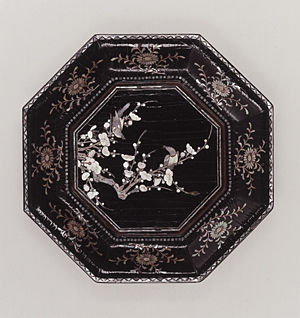The image depicts a small, square, octagonal dish with a light gray background and no border or text. The outer rim of the dish is silver, transitioning to a dull gray, giving it a metallic appearance. This outer section encircles a black layer adorned with a silver floral pattern, adding elegance to its design. The center of the dish features another black octagonal area, where white, branch-like patterns with small leaves stretch from the left side across to the right, enhancing its decorative appeal. The entire dish reflects light subtly, emphasizing its delicate and possibly expensive craftsmanship.